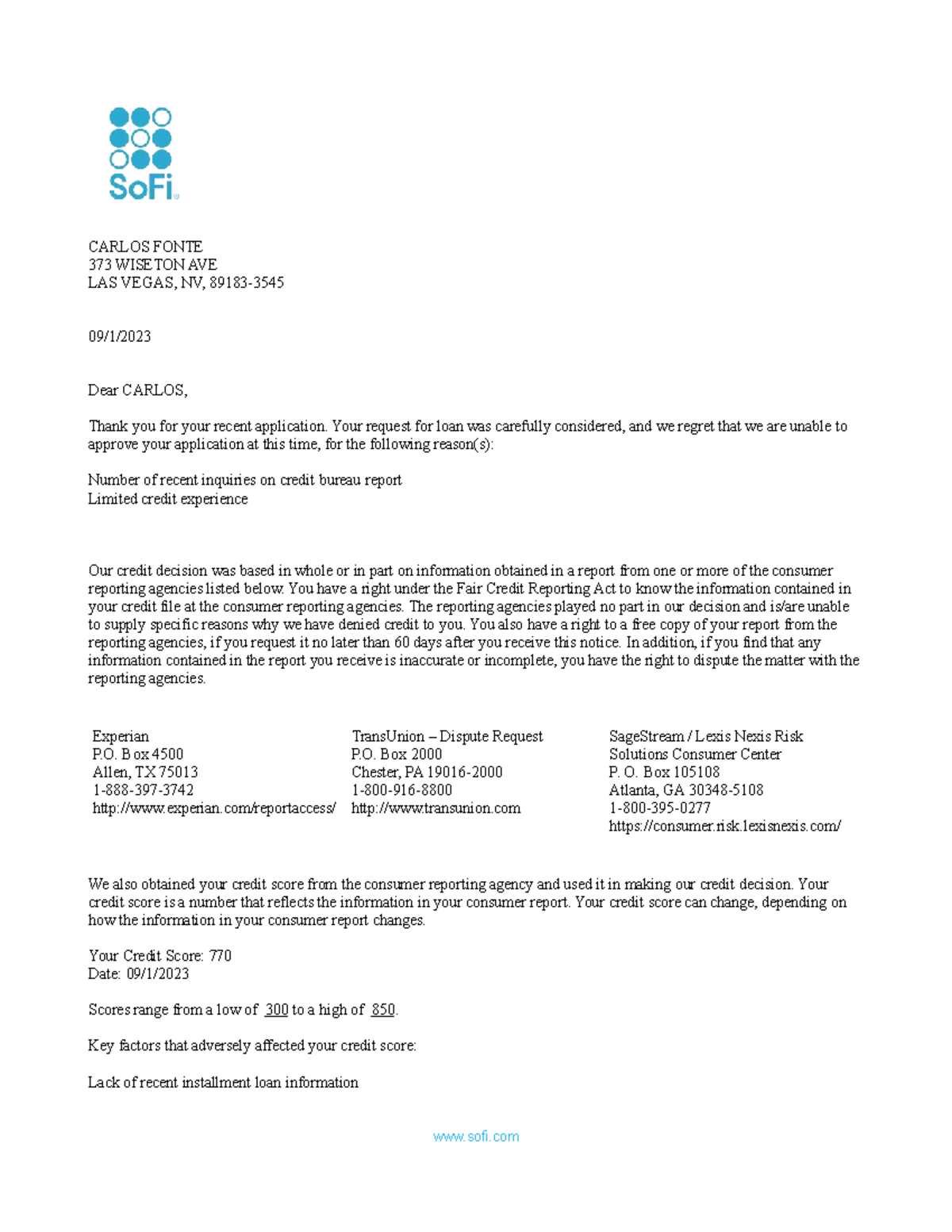Screenshot of a rejection letter received via email from SoFi. In the upper left-hand corner, the sender is identified as SoFi. The letter is addressed to Carlos Fonte at 375-3 Wisetown Avenue, Las Vegas, Nevada, 89183. The letter begins with a salutation, "Dear Carlos," and proceeds to thank him for his recent loan application. It states that his loan request was carefully considered but ultimately declined. The letter goes on to provide detailed reasons for the denial, including specifics about his credit score and other relevant information. This document serves as an official notification of the loan rejection.